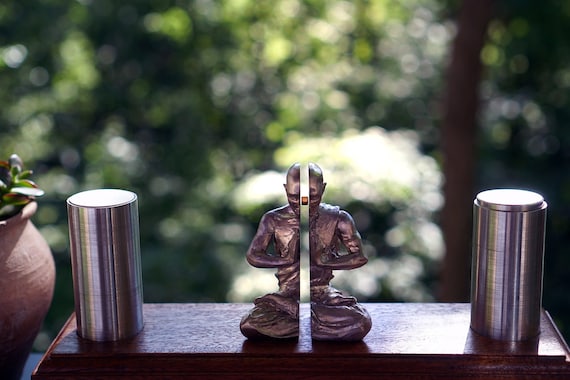The photograph captures a close-up of a serene garden scene, likely set on a table or shelf. Central to the composition is a bronze Buddha statue, posed in a meditative posture with its legs crossed and hands clasped together. The statue features a striking silver stripe running from its head down to its folded feet, and it appears to function as a bookend, as one half is visible in the frame. Flanking the statue are two tall, silver cylindrical objects. In the backdrop, a lush garden is partially visible, with sunlight dappling the green bushes and tree trunks behind. Adding to the tranquility are white flowers and a prominent reddish-brown vase containing green lettuce plant leaves, contributing to the overall meditative ambiance of the scene.